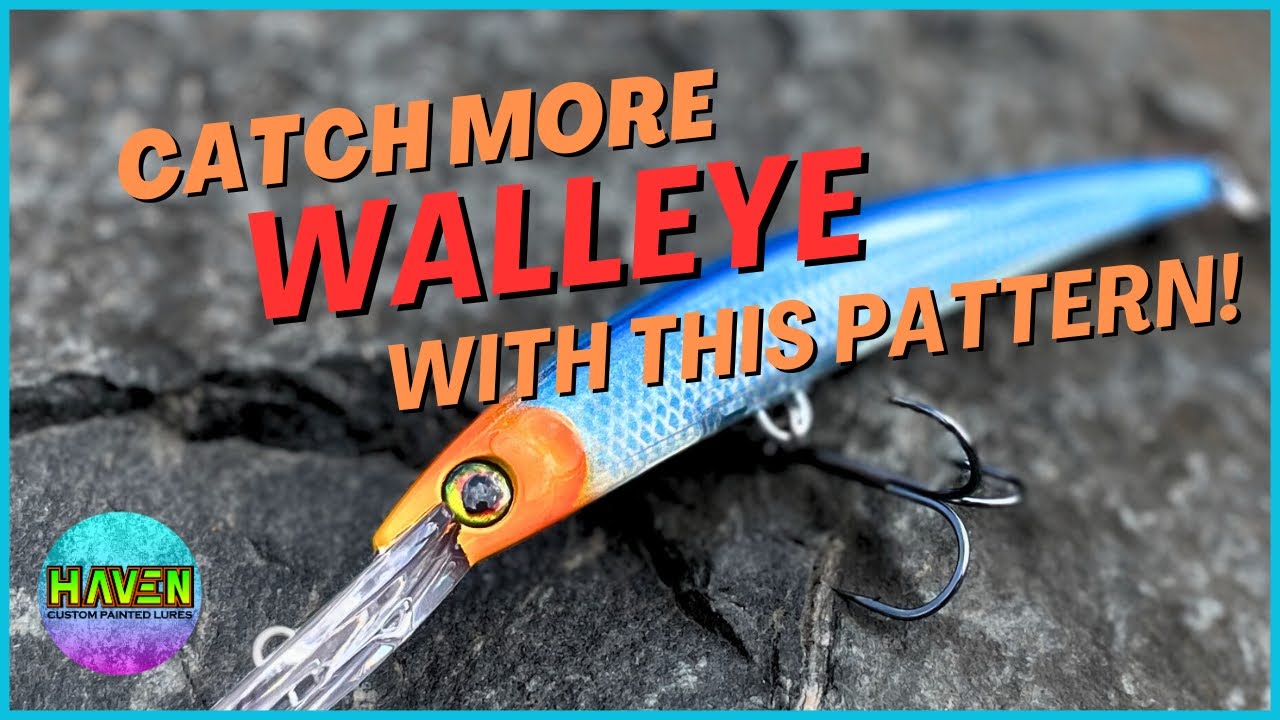The image is an advertisement for a fishing lure named "Haven Custom Painted Lures." The background shows a large flat gray rock, resembling asphalt or granite, with a prominent crack extending from the left-hand side. Overlayed on the rock are bold, capitalized letters in vibrant colors. The text reads, "CATCH MORE WALLEY" in large red letters and "WITH THIS PATTERN" in smaller orange letters. At the bottom left corner, there's a circular logo displaying the company's name, "Haven Custom Painted Lures."

The lure itself is prominently featured in the center of the image. It has a shiny, almost metallic blue body, transitioning from royal blue along the spine to lighter blue on the sides. The head is bright orange, and the lure has a striking yellow and black eye. Emerging from its mouth are clear, flexible vinyl tendrils. Attached to the underside of the lure is a dark silver, nearly black, three-pronged hook. The vivid lure and the rugged rock background create a visually impactful advertisement aimed at anglers looking to catch more walleye. The entire image is bordered by a light, possibly teal, frame, adding a finishing touch to the ad.